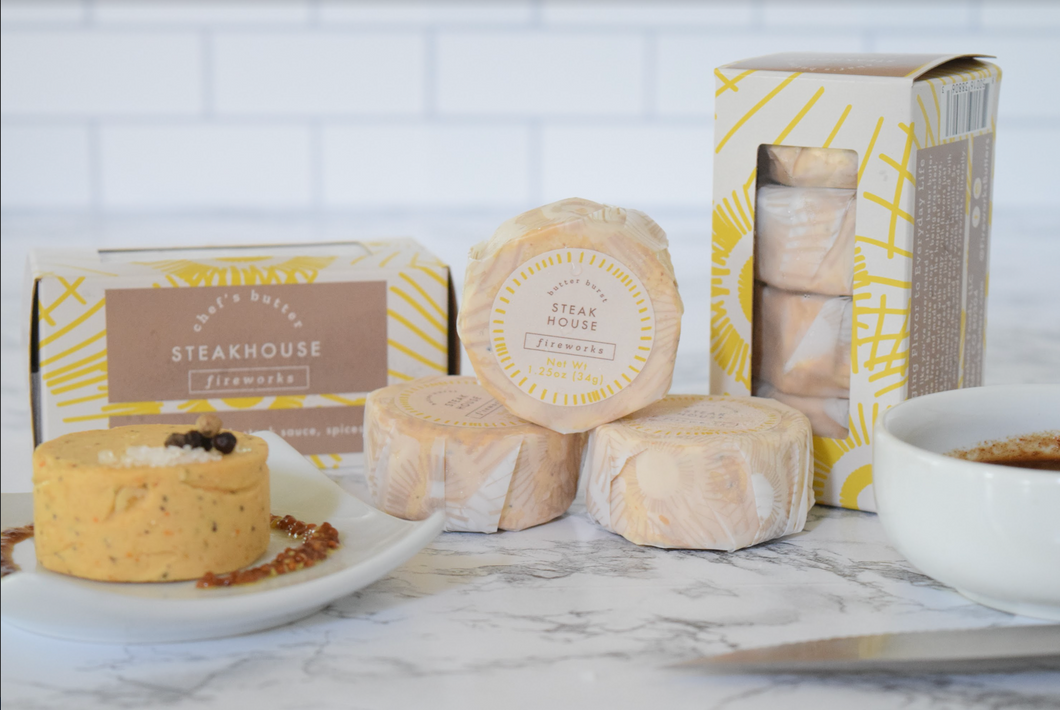In an indoor kitchen setting with a white marble countertop accented with gray, the photo displays a detailed arrangement of food items backed by a slightly blurry, white tiled wall. Central to the image is a white china plate that holds a thick, circular yellow and orange patty called Chef's Butter Steakhouse Fireworks, with black garnish on top and a red garnish drizzled on the side in an elaborate pattern. Surrounding this plate are three additional patties wrapped in wax paper, two lying flat and one standing upright facing forward, labeled "Butterburst Steakhouse Fireworks, net weight 1.25 ounces, 3.4 grams." Next to them is a box matching the wrapped patties, featuring a transparent side that reveals four more patties inside. The box is predominantly white with yellow streaks and brown labeling that reads "Chef's Butter Steakhouse Fireworks." To the right sits a white bowl containing a brown condiment, possibly a sauce, partially visible due to the frame's angle. The entire setup is artfully arranged on this grey-streaked white marble countertop with the backdrop of a white brick wall, suggesting a modern and sleek culinary environment.